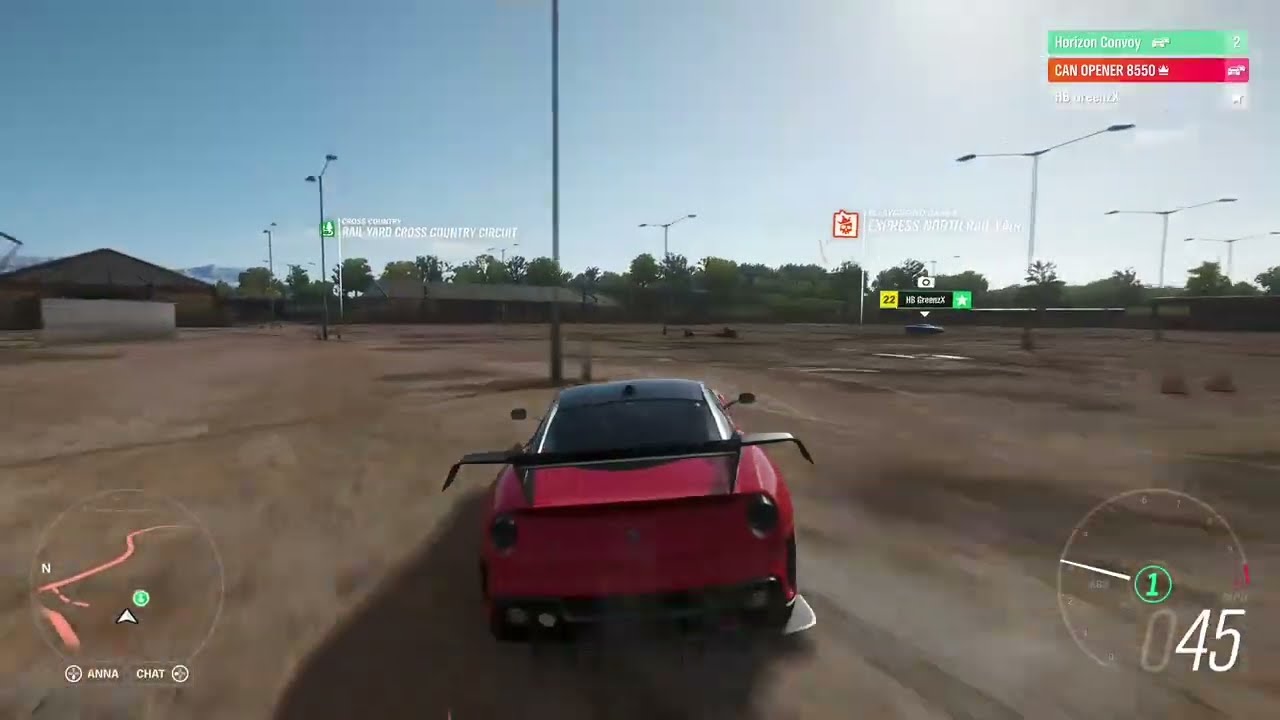This screenshot captures a vivid scene from a new-generation video game, likely a racing simulator. Dominating the foreground is a sleek red sports car, viewed from behind as it appears to speed away on a bare dirt surface, casting a shadow beneath it. The car features a black roof and a black spoiler, with dark red taillights and a black bumper. In front of the car, the ground is dotted with a few mud puddles, while the surrounding setting resembles a sprawling parking lot. 

The sky above is a striking blue, punctuated by the bright sun and occasional clouds. Multiple light poles are scattered throughout the area, complete with lamps casting light in different directions. In the background, a line of green-leaved trees and a collection of large metal buildings with arched roofs can be seen.

The game interface is also visible: the upper right corner displays two banners with the text "Horizon Convoy" in green and "Can Opener 0550" in red. A detailed radar-style map is located in the bottom left corner, featuring a pink path and the letter 'N', along with the word 'Anina' and a 'Chat' option. The bottom right corner shows a speedometer marked with the number 1 in green, with additional numerical details highlighted in different colors.